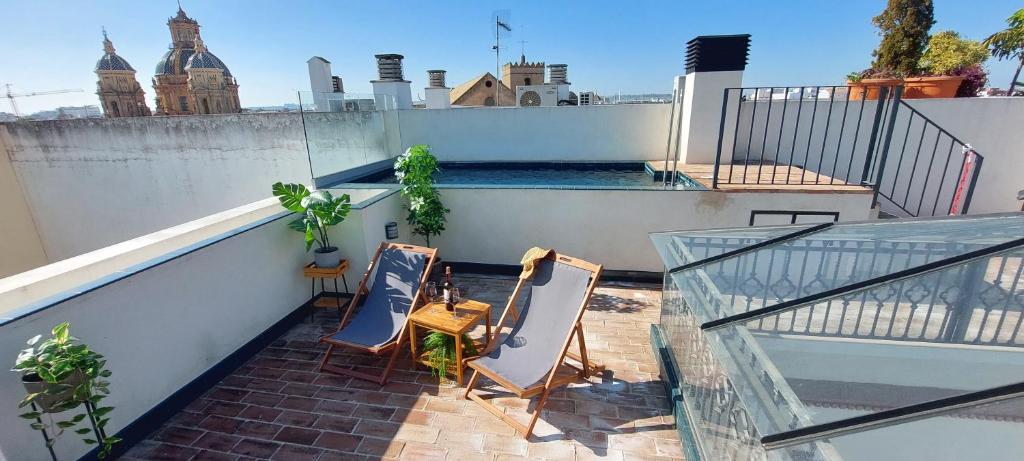The professionally taken image captures an inviting rooftop patio, adorned with reddish-brown brick flooring and enclosed by a white half wall. Dominating the scene are two wooden, fold-up chairs with canvas seats, positioned side by side, accompanied by a small wooden table between them. The table is set with two wine glasses and a bottle of red wine, hinting at a leisurely afternoon. A potted plant graces the lower left corner of the image, adding a touch of greenery. On the right side, a large skylight bathes the area in natural light. The backdrop reveals a banister and a panoramic view of majestic, possibly cathedral-like buildings, with trees contrasting against a vivid blue sky. In the distance, there's a suggestion of a swimming pool accessible by a small set of stairs. The color palette features a harmonious blend of black, white, gray, green, brown, terracotta, and red, creating a tranquil and picturesque setting without any text to distract from the visual elements.